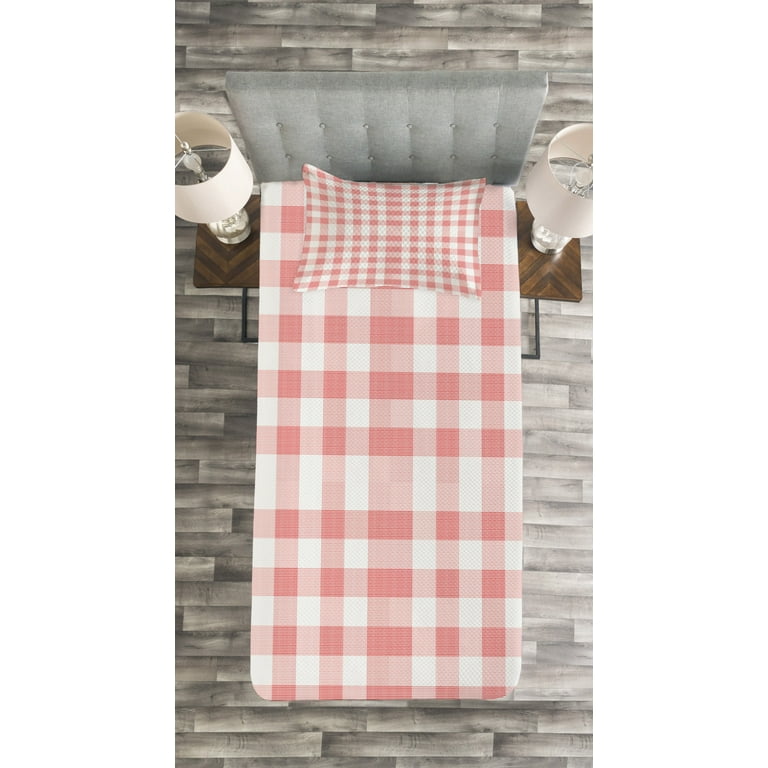This image, taken indoors, features a top-down view of a single or twin-sized bed, which dominates the composition, suggesting an intimate and cozy setting. The backdrop appears almost computer-generated, enhancing the aesthetic with a modern, stylized ambiance. The bed's headboard is a gray, textured, and ruffled button cushion, adding a touch of elegance. Flanking the head of the bed are two wooden nightstands with black metal bases, each adorned with a single cylindrical, white lampshade lamp. The bed itself is dressed in a pink and white plaid pattern, with a pillow at the head featuring a tighter, matching plaid pattern. The floor and adjacent wall both feature a grayish-brown wood design, blending seamlessly to create a harmonious and inviting space.